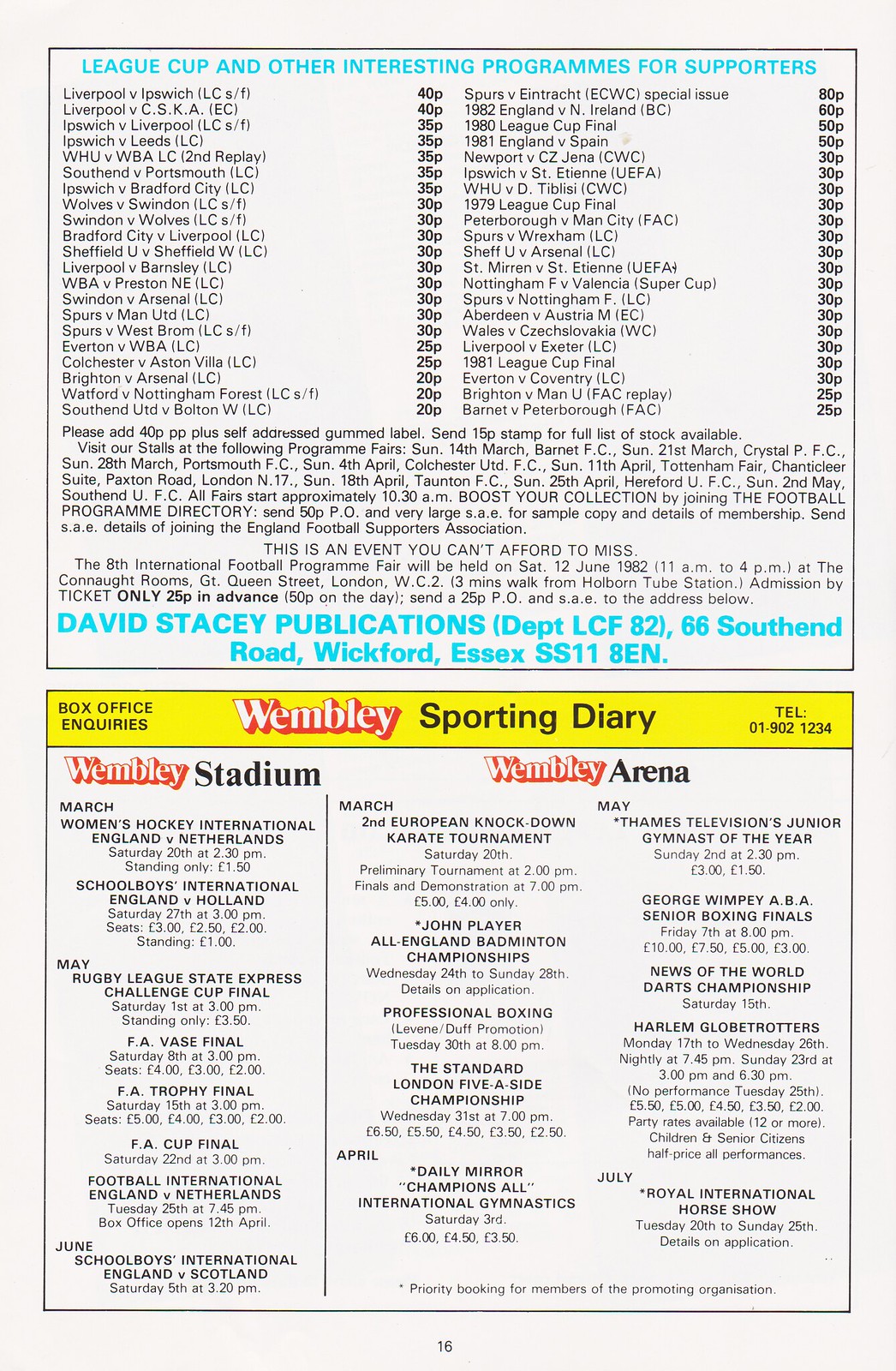The vertically aligned rectangular image showcases a printed sheet of paper bordered by a thin black line. At the top, in blue text, the title reads "League Cup and other interesting programs for supporters." The middle section provides detailed match-ups of various sports teams listed in two columns, ranging in price from 20p to 80p. For instance, match-ups include "Liverpool versus Ipswich, 40p" and "Spurs versus Untracked ECWC special issue, 80p." Additional textual information includes, "David Stacey Publications, DEPTLCF82, 66 South End Road, Wickford, Essex, SS118EN," along with directives to "please add 40p plus self-address gummed label" and "send 15p stamp for full list of stock available."

The bottom section prominently features a yellow banner with red text stating, "Wembley Sporting Diary," and includes a line for "Box Office Inquiries, Telephone 01-902-1234." Beneath this, against a white background, are two columns headed "Wembley Stadium" and "Wembley Arena." The "Wembley Stadium" column details upcoming events such as March Women's Hockey International: England versus Netherlands, School Boys International: England versus Holland, and notable finals like the FA Vase Final, FA Trophy Final, and the FA Cup Final. The "Wembley Arena" column lists events such as the March 2nd European Knockdown Karate Tournament, John Player All England Badminton Championships, and Professional Boxing, followed by other events available for spectators.